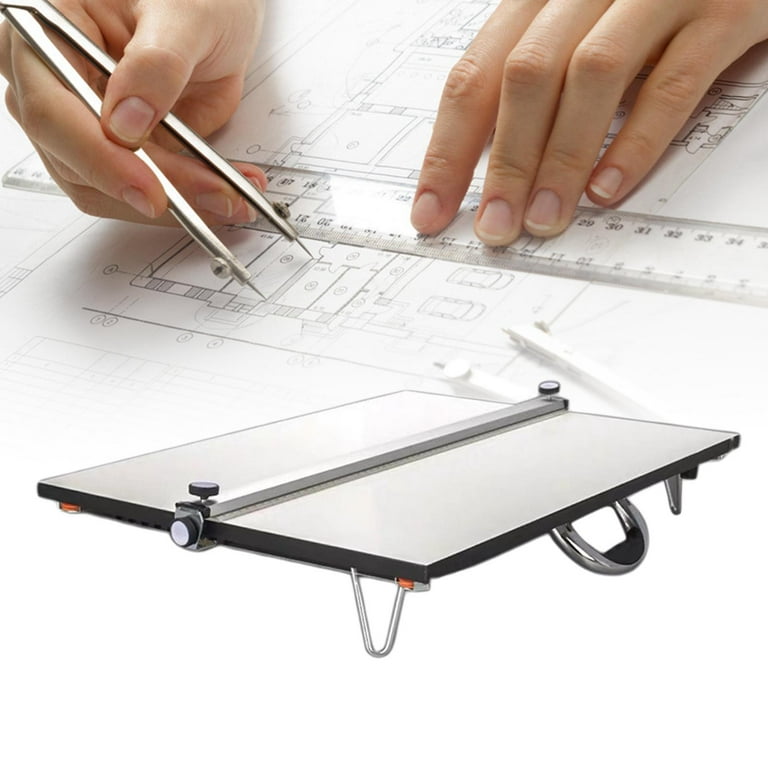This color photograph features a meticulous drafting scene. At the top of the image, a pair of hands of indeterminate gender, with short and neat nails, are engaged in precise measurement tasks. The left hand grasps a metal protractor, and the right hand steadies a clear ruler. These tools are being used on a large sheet of paper filled with different drafting elements, diagrams, and what looks like a building floor plan, including outlines indicative of two vehicles. Below this drafting activity, the photograph showcases a metallic item whose function is unclear. This object is a silver metal rectangle with a rectangular prism in the center, secured by two black bolts. Additionally, it features a silver hook extending from the front side and another protruding from the middle, suggesting it might be part of a measurement or placement tool potentially used in the context of blueprint analysis. The precise purpose of this metal item remains unidentified without further context. There is no text in the image to provide additional clues.